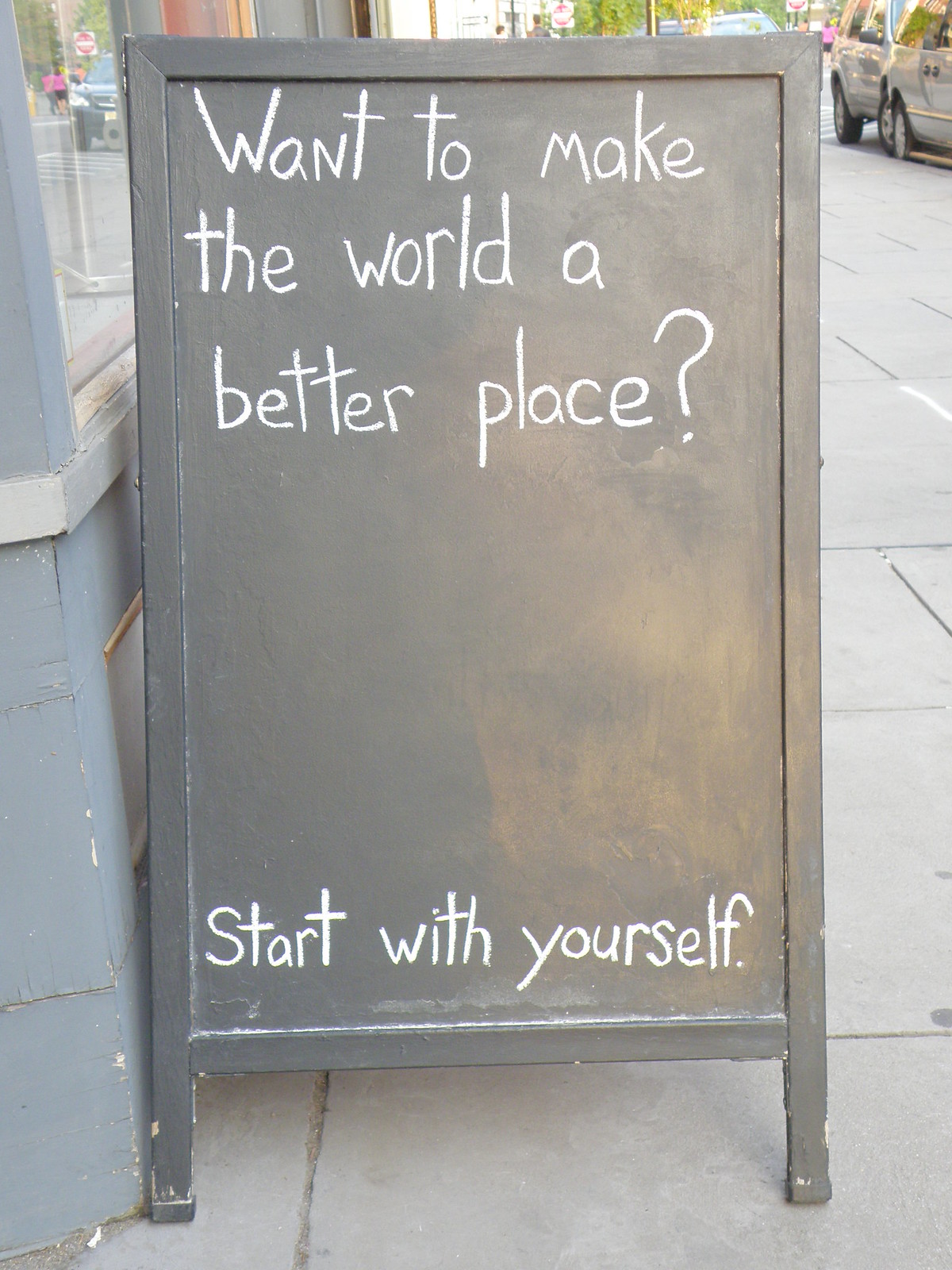The image captures a simple yet impactful scene on a city sidewalk right outside a storefront or restaurant. The main focus is a black framed, wooden chalkboard sign painted with a dark gray or black finish, placed prominently on the sidewalk. In striking white chalk, the sign displays a motivational message: "Want to make the world a better place? Start with yourself." This handwritten message is clearly legible and remains the central element of the photo. In the background, there are a few cars parked along the sidewalk and the building adjacent to the sign features blue-painted bricks and a large glass window, suggesting a friendly business environment. The scene is set against a backdrop that includes hints of green, possibly from trees, although details about the broader setting and any passersby are not visible.